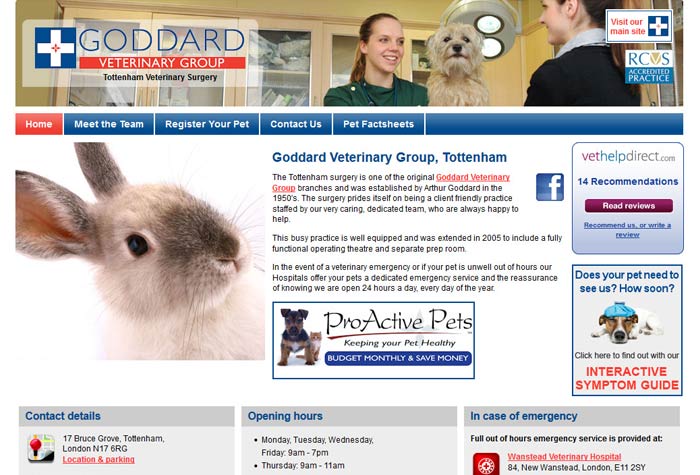This image is a detailed screenshot of the home page of a website for a veterinary group. The header at the top of the page features a captivating photo: on the far left, large blue capital letters spell out "Goddard" against the background. Adjacent to this, there's a narrow red rectangle with white text that reads "Veterinary Group." Below this is smaller text stating "Tottenham Veterinary Surgery." To the left of this text is a blue square with a white cross symbol.

The central part of the header contains a photograph displaying a young white woman, likely in her early 20s, with reddish-brown hair neatly pulled back behind her ears, smiling warmly. She is accompanied by a very shaggy dog with almost white, slightly grayish fur. On the right side of the header, a side profile of another white woman wearing a black shirt is partially visible.

Beneath the header is a navigation menu. The leftmost item, set against a red background, is labeled "Home." The remaining menu items are set against a blue background and are labeled in white font as "Meet the Team," "Register Your Pet," "Contact Us," and "Pet Fact Sheets."

Further down the page, on the left side, there is an image of a rabbit's head with very light gray fur, slightly darker around the nose and ears. On the right side of this image, a headline in blue font reads "Goddard Veterinary Group, Tottenham." Beneath this headline, a description in red underlined text, indicating it is likely a hyperlink, states, "The Tottenham Surgery is one of the original Goddard Veterinary Group branches and was established by Arthur Goddard in the 1950s. The surgery prides itself on being a client-friendly practice staffed by our very caring, dedicated team who are always happy to help." This description continues further below.

On the right side of the page, there is a light blue square featuring a likely advertisement from "help direct.com," which notes "14 recommendations." Below this ad, a maroon rectangle with white text prompts visitors to "Read Reviews."